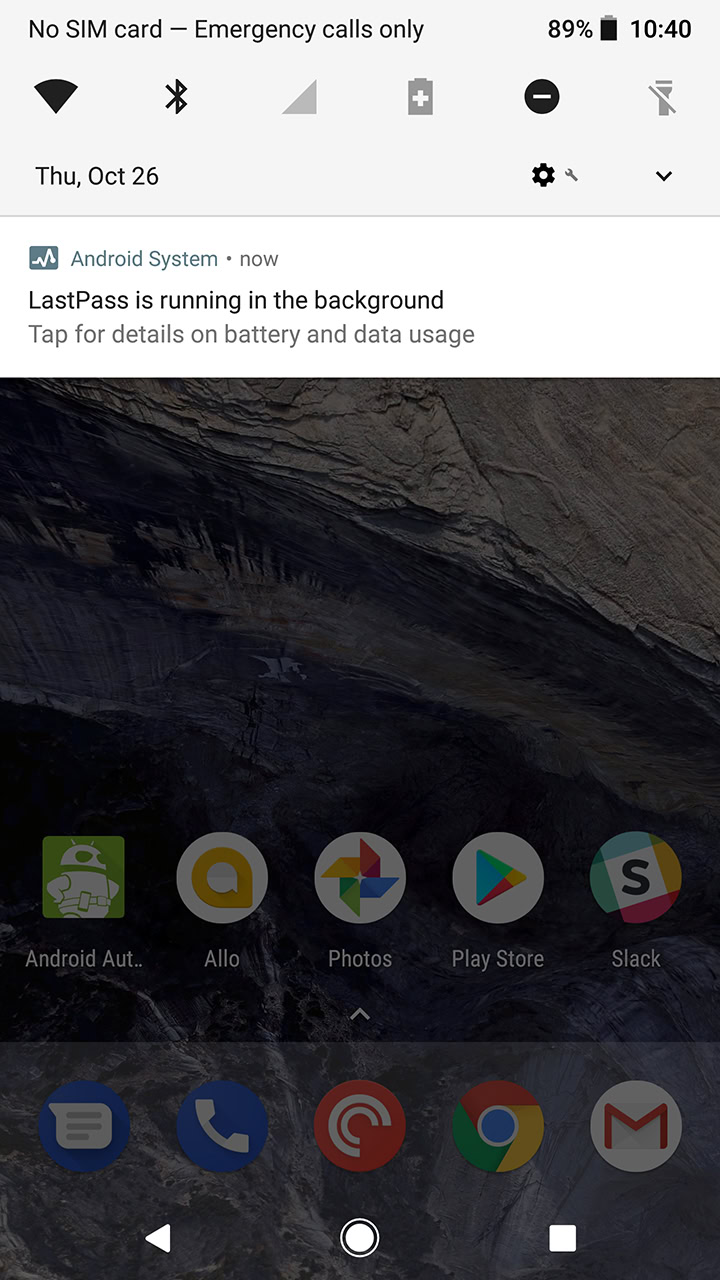A detailed screenshot of a cell phone's status bar and notification panel is depicted. In the upper left-hand corner, black text reads "No SIM card, emergency calls only," indicating that the device isn't connected to a cellular network. On the upper right-hand side, the battery life is displayed as "89%." The current time shown on the screen is 10:40. Directly beneath this, various icons are lined up, including the Wi-Fi icon, Bluetooth icon, cell phone reception icon, battery icon, "Do Not Disturb" icon (circle with a horizontal line in the middle), and the flashlight icon. Notably, the flashlight icon, battery icon, and cell phone reception icon are grayed out, signaling that these functions are either inactive or unavailable.

In the top information bar, the date is listed as "Thursday, October 26" in the lower left corner of this section. To the lower right of this same section, there is a settings icon alongside a drop-down arrow icon, hinting at additional options or settings that can be accessed.

Below this information bar, a white notification block appears with the title "Android system." The block contains a notification from LastPass, stating, "LastPass is running in the background. Tap for details on battery and data usage," providing an alert regarding the app's operational status and resource consumption.